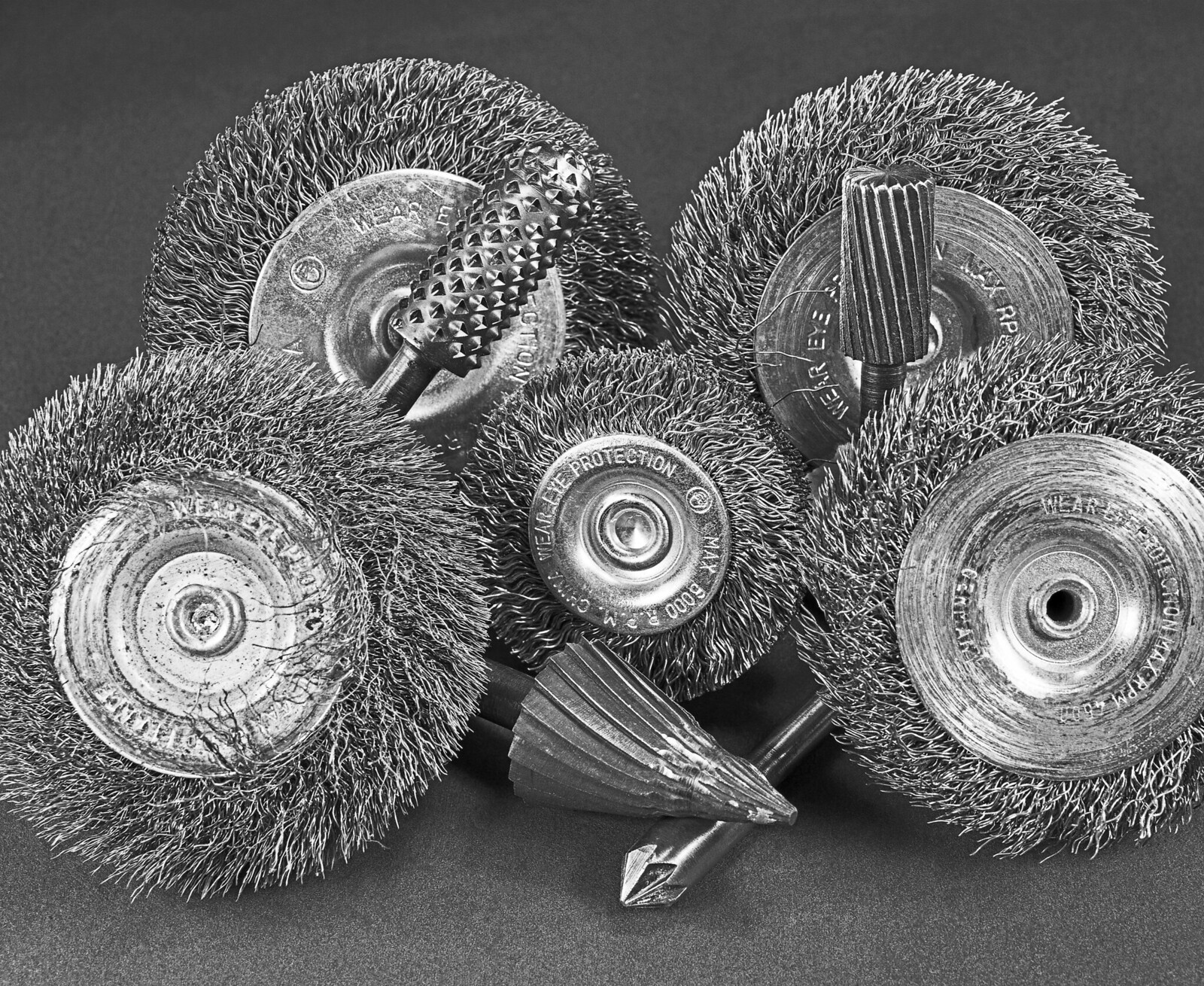This black-and-white photograph has an intriguing surreal quality, resembling a piece of AI-generated art. The image captures five large metallic wheels arranged in a diamond-shaped pattern, with the central wheel being slightly smaller than the surrounding ones. Instead of traditional tires, the wheels have bristle-like grass growing outwards, all oriented to the right. 

The wheel on the left features a large, conical metallic implement with a texture that resembles sheaf grass. Similarly, the wheel on the upper right has a conical attachment with diagonal lines etched onto its surface. Positioned just below the central wheel on the floor is another conical implement, distinguished by lines that run from its tip to its base and a top that appears slightly bent or crushed. Underneath this, there is a long metal spike, tapering towards one end before expanding into a diamond shape, reminiscent of a pencil.

All of these elements are set against a textured grey background, with the floor visually distinct from the darker wall behind it. Upon closer inspection, the wheels reveal shiny silver parts with inscriptions and include a directive to "wear eye protection," accompanied by a date of May. Scattered among the wheels are various black and silver metal pieces, some adorned with lines and others with pokes and grooves, adding to the intricate, otherworldly aesthetic of the scene.